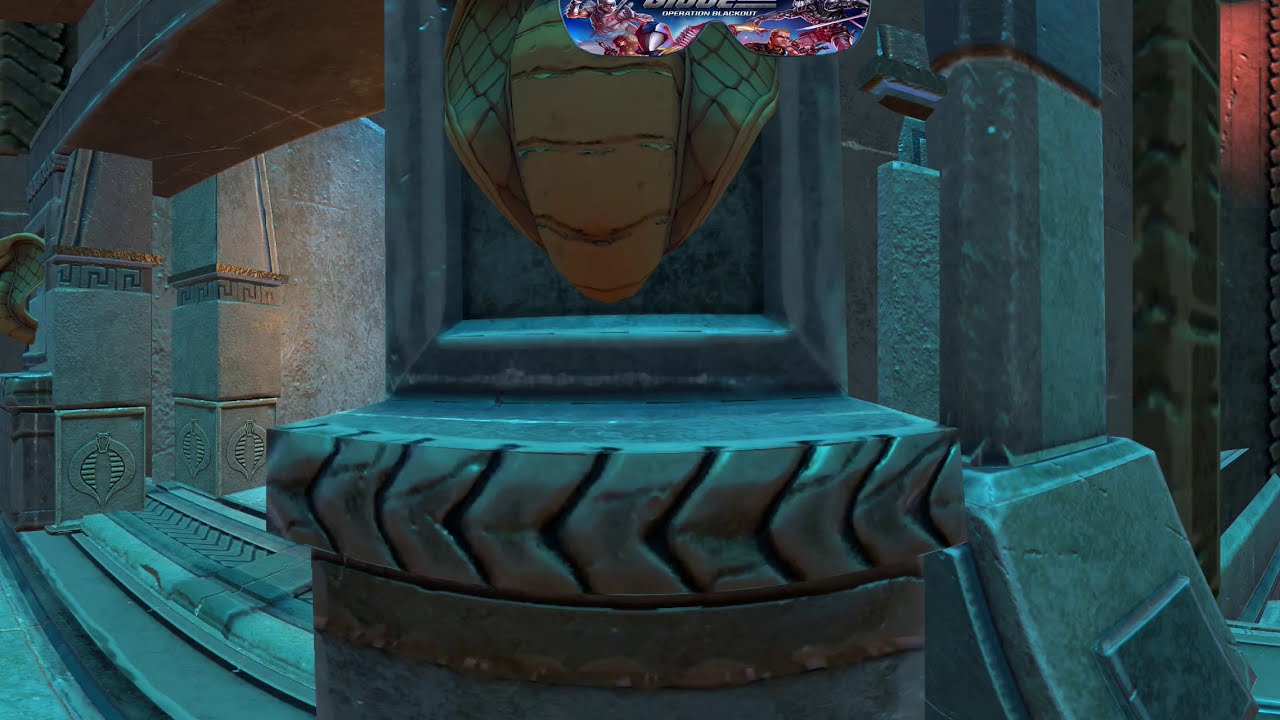The image appears to be a detailed scene from a video game, set in a dungeon-like temple with a mystical atmosphere enhanced by a bluish hue. Central to the image is a stone pillar, adorned with a framed, golden object that resembles a stylized depiction of a winged creature or possibly a piece of ornate plate mail. This frame resides in what looks like an indented oval setting. Above the frame, a banner or in-game advertisement reading "Operation Blackout" stretches across the image, decorated with characters that give off a GI Joe vibe.

To the left of the pillar, there are stone steps ascending to a passageway that disappears from view, suggesting further exploration. Nearby, stone walls and carved columns display images of cobra heads, emphasizing the temple's serpentine theme. Below the centerpiece, a cylindrical stone base with possible tire tread-like imprints extends downwards, its full length cut off by the edge of the image. 

On the right, another hallway extends, framed by more intricately carved stone columns, while to the left, an adjoining room hints at additional cobra statues. The overall feeling is one of an ancient, fantastical environment, meticulously crafted for an immersive gaming experience.